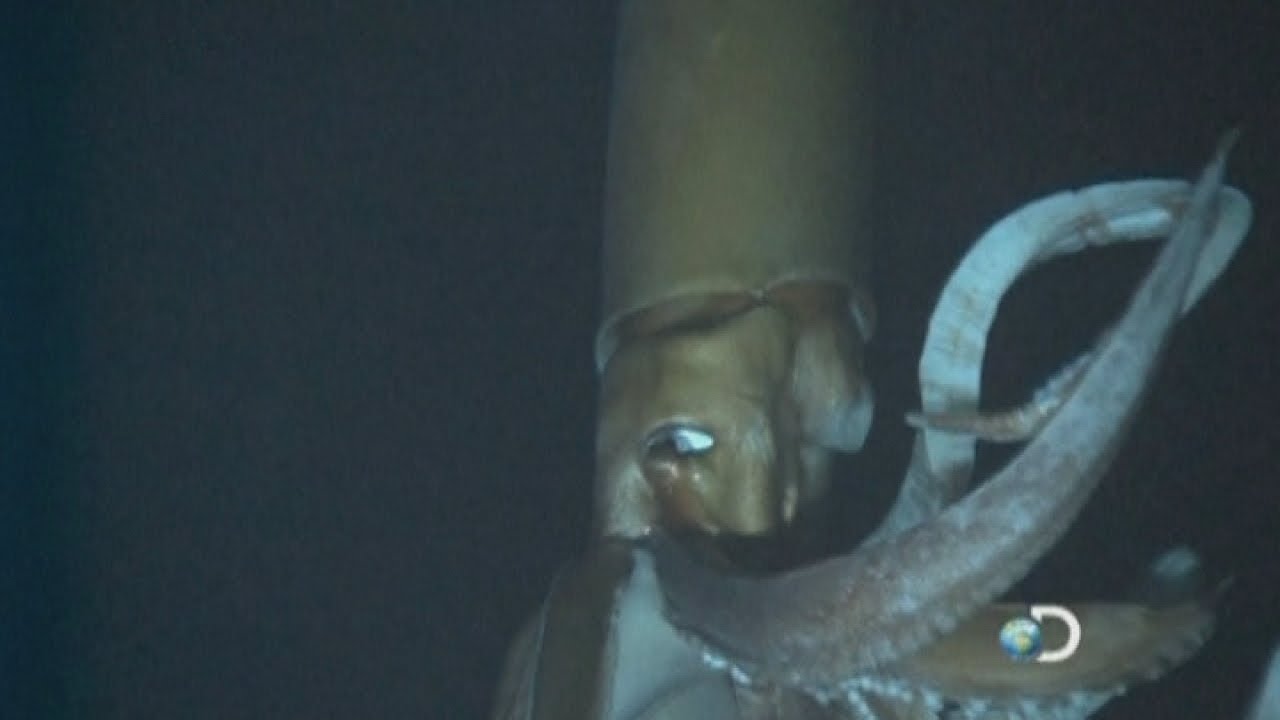This landscape-oriented photograph, possibly a nighttime TV program screenshot from the Discovery Channel, features a blurred close-up of a large octopus in dark ocean waters so deep they appear almost black. The octopus, predominantly brownish with some light teal blue markings on its tentacles, occupies most of the right side of the image. It has wide-open eyes seemingly looking at the camera, although the blurriness makes it hard to tell for certain. The tentacles are visibly swinging, adding a sense of dynamic motion to the scene. In the bottom right-hand corner, the Discovery Channel logo, consisting of a capital 'D' interwoven with a globe, is clearly present. Amidst the blurry details, there's also a faint, indistinguishable human face visible within the composition.